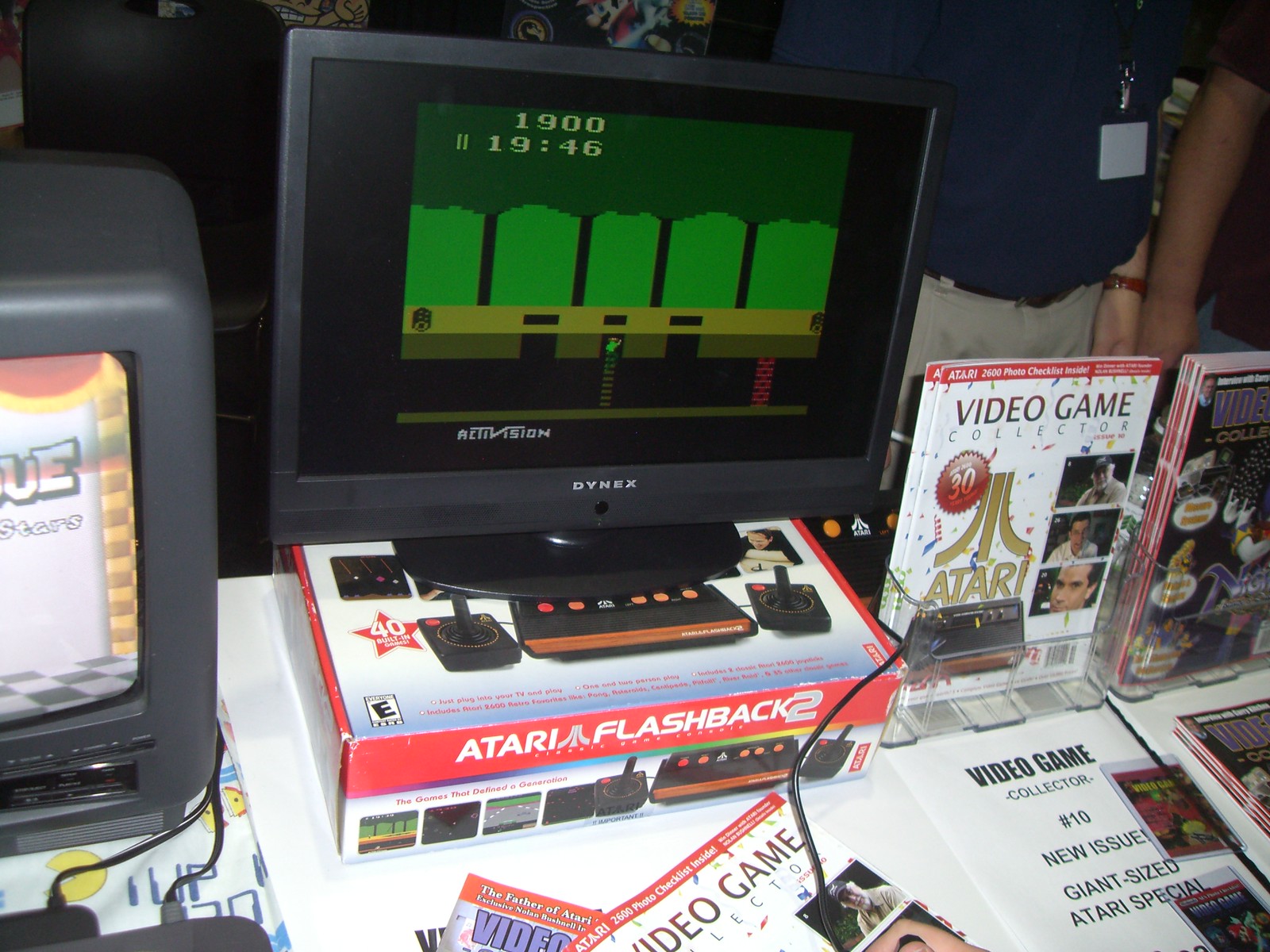The photograph showcases a nostalgic gaming setup at what appears to be a convention. Central to the image is a gray Dynex flat-screen monitor displaying an early 90s, pixelated video game characterized by a brick top, pixelated graphics, and a brown ground at the bottom third of the screen. This monitor sits atop an Atari Flashback 2 box adorned with colorful images of classic game screenshots and marked with an "E for Everyone" logo. In front, there are video game magazines scattered on the countertop, including one prominently featuring "Video Game Collector," advertising a giant-sized Atari special issue. Adding to the retro ambiance, to the left, there's the partly visible screen of an older black CRT TV with black wires connecting to it. Clear stands used for displaying prints and magazines are also evident. In the background, partially visible are the torsos of two individuals, one wearing a dark blue shirt and khaki pants, and the other a reddish shirt and an ID tag on a lanyard, further hinting at a convention setting.